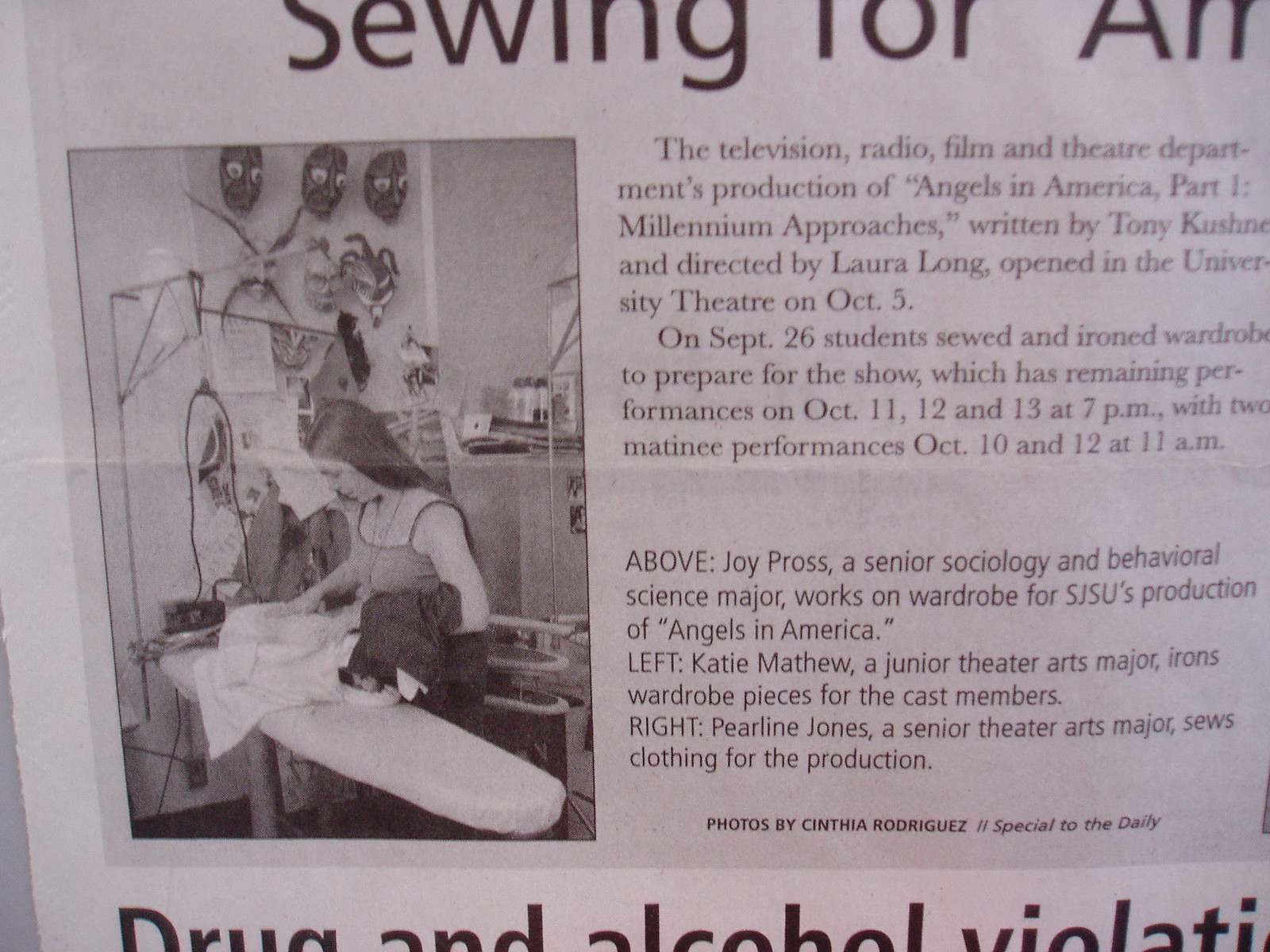In a black and white photo taken from a newspaper or magazine, the central image is of Katie Matthew, a junior theater arts major, diligently ironing wardrobe pieces for SJSU's production of "Angels in America, Part One: Millennium Approaches," written by Tony Kushner and directed by Laura Long. The production, overseen by the Television, Radio, Film, and Theater Department, opened in the University Theater on October 5th, with performances continuing on October 11th, 12th, and 13th at 7 p.m., and matinee shows on October 10th and 12th at 11 a.m. Accompanying Katie in the wardrobe department are Joy Pross, a senior sociology and behavioral science major, and Caroline Jones, a senior theater arts major, both contributing to the creation and preparation of costumes. The caption reveals that the photo session capturing these moments took place on September 26th. The photo credit goes to Cynthia Rodriguez, and a note at the bottom of the image mentions drug and alcohol violations.